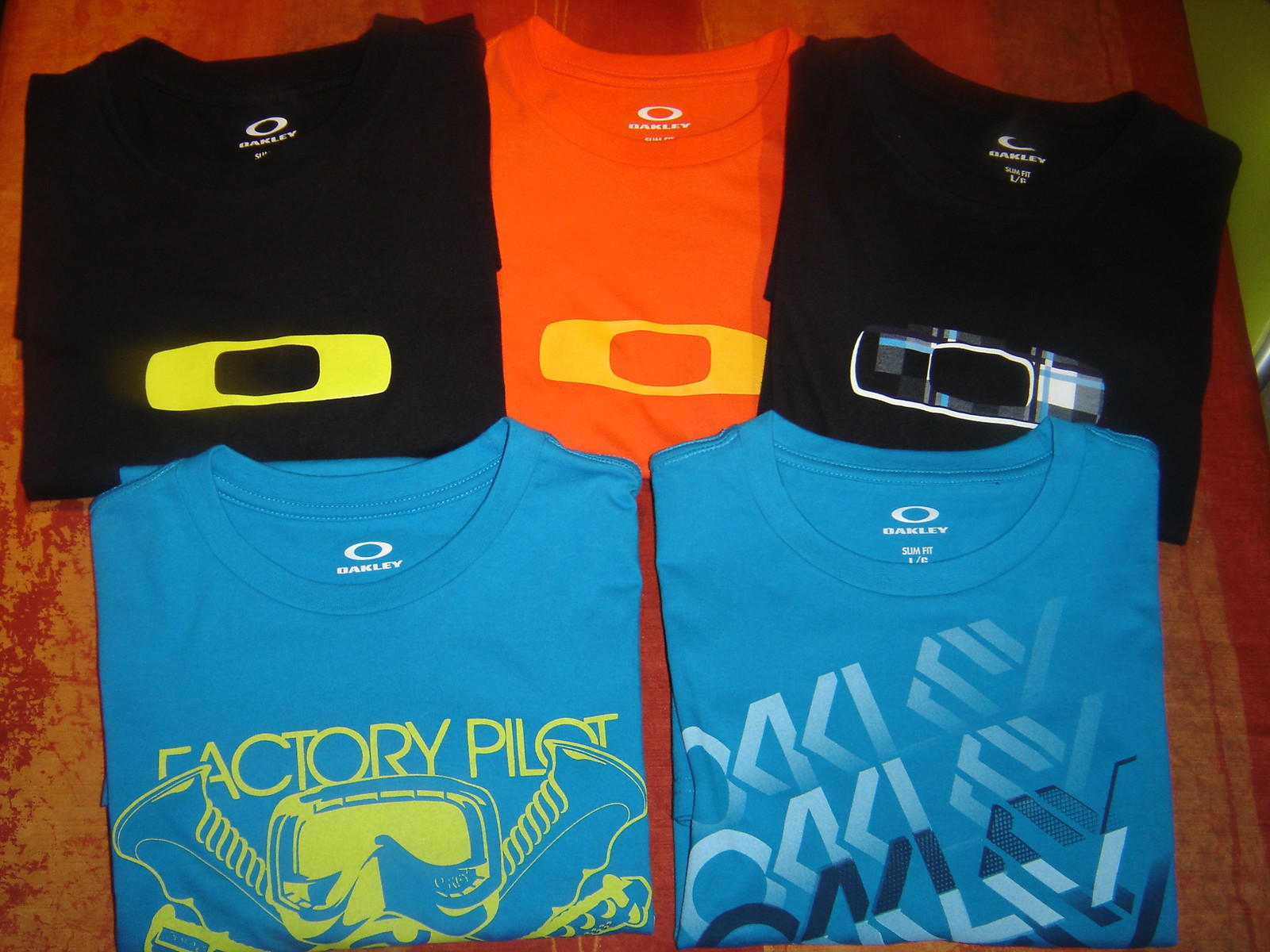The image showcases five neatly folded Oakley t-shirts arrayed against a mottled red fabric background. Each shirt bears the Oakley logo prominently. Starting from the top left, there's a black t-shirt featuring a large yellow "O" in the center. The middle shirt in this row is a solid orange with the same yellow "O" symbol centered on its front. On the top right, another black t-shirt displays a distinctive blue and white 'O' design with a plaid-like pattern. 

The bottom left shirt is blue and carries the phrase "Factory Pilot" in yellow lettering, accompanied by an image that resembles a face mask in the same yellow. The final t-shirt on the bottom right is also blue, marked with the Oakley brand name in varying shades of blue and white, cascading down the front. All the t-shirts are arranged meticulously, providing a clear view of their front designs.